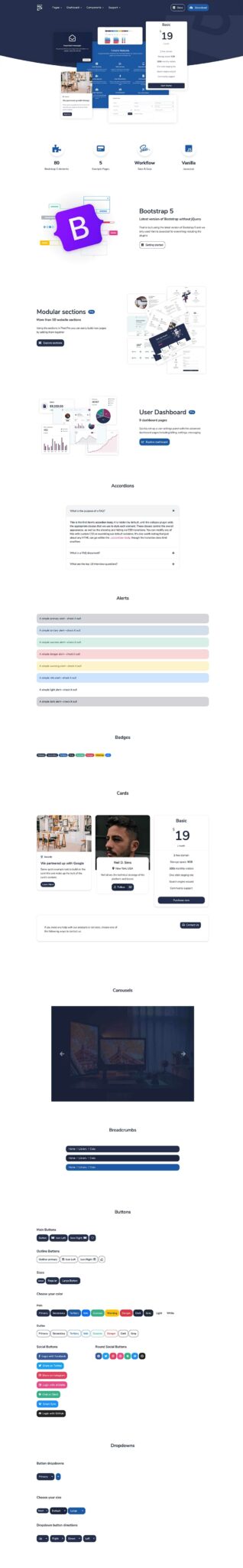A long and blurry screenshot of a complete web page, seemingly designed to simulate the experience of scrolling through it. The page features a predominantly white background with a dark navy blue header at the top, which is rectangular with a downward curve towards the center. The layout includes multiple large images interspersed with text beneath them. Rows of pastel-colored text in shades of gray, light green, pink, and peach also appear, adding a soft, inviting visual element. Further down, more images paired with text are visible, along with various colorful accents spread throughout the page, demonstrating a diverse and lively web design.